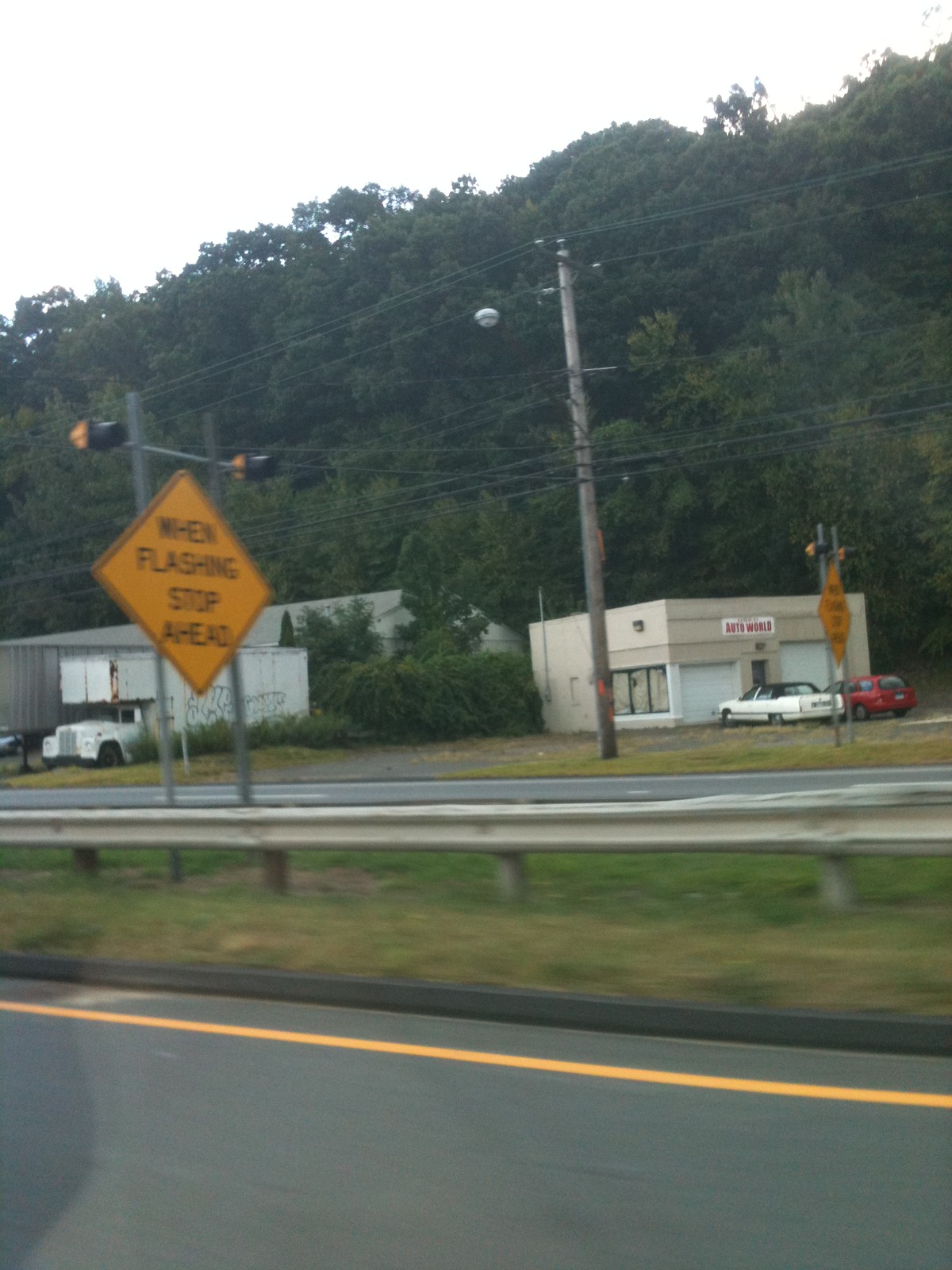The image captures the side of a highway, featuring a guardrail adjacent to a grassy divider. Prominently displayed is an orange diamond-shaped traffic sign that reads "When Flashing Stop Ahead," flanked by two yellow lights on its upper corners. The highway's dark gray pavement is marked with a yellow line running horizontally. In the background, several telephone poles stand amongst lush, overgrown greenery and large trees that dominate the landscape. Amidst the foliage, an auto parts store named "Auto World" is visible, along with a red station wagon and a white Cadillac. To the left, there's an old box truck, adorned with graffiti, that appears to be abandoned. These details paint a vivid picture of a somewhat retro, rural roadside scene, blending natural and man-made elements.